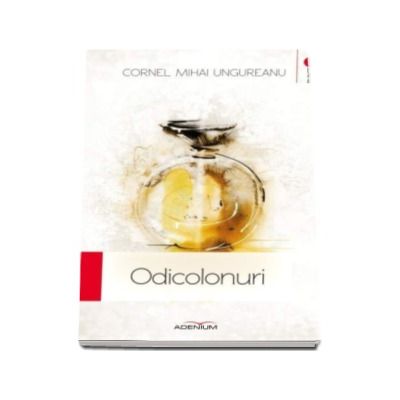The image features a low-resolution depiction of what appears to be an advertisement or book cover related to a fragrance, placed against a pure white background. At the top, in gray text, it reads "Cornell Mihaly Unger-Reneau." Below this, there is a clear, oval-shaped glass bottle with a round cylindrical stopper, containing a yellow liquid, likely representing a perfume. The bottle is depicted in a style that suggests it could be a painting or a detailed illustration. Directly beneath the bottle, in slim type, possibly gray, is the word "Odikolonuri," with a small vertical red rectangle adjacent to it on the left side. At the very bottom, there is black text indicating the publisher, "Edenium," which also features small red wings over the letters "N" and "I." The entire design is framed within a vertical rectangle, emphasizing its advertisement-like layout, or possibly a book cover, all set against a clean white background.